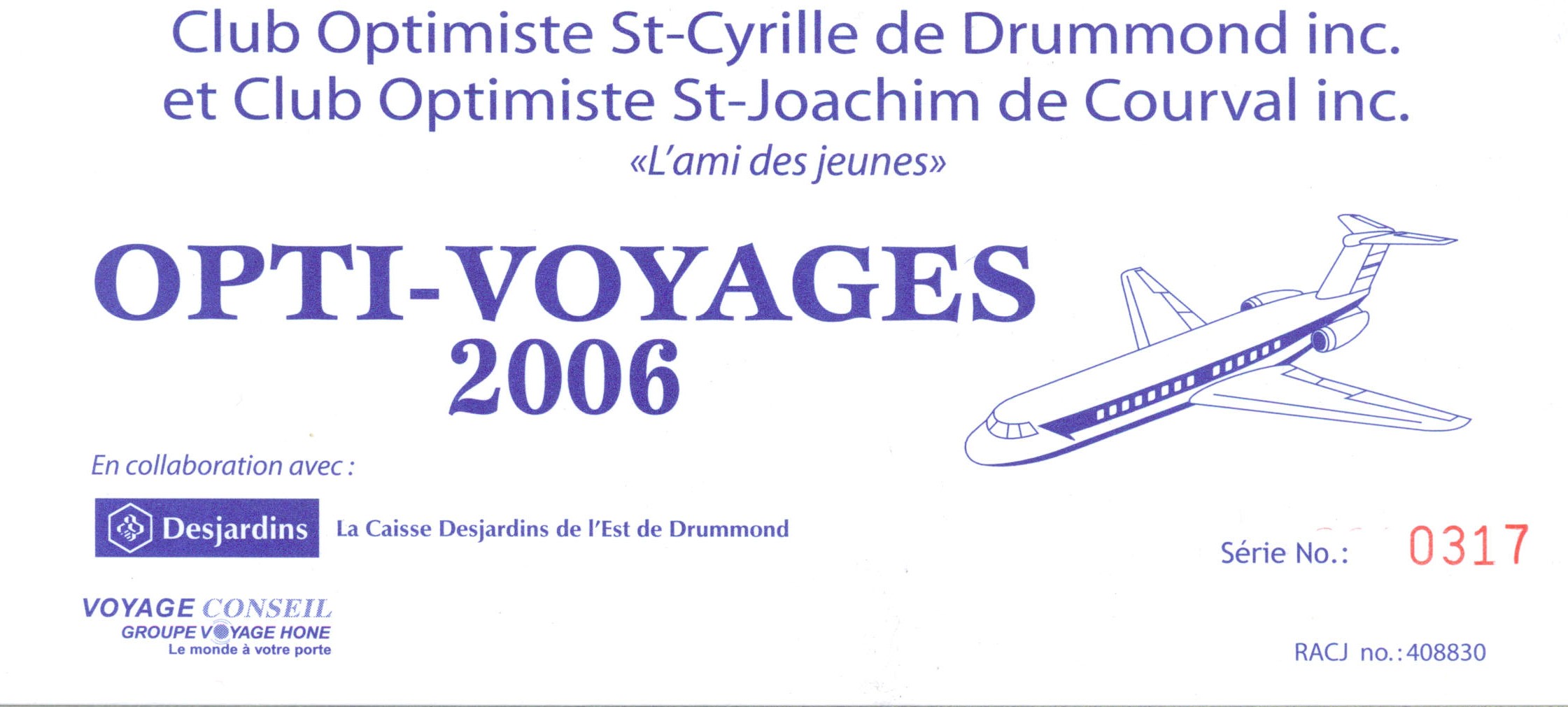This is an advertisement for an airline company, primarily written in French, set against a white background with blue print. At the center of the piece is a detailed sketch of a very large aircraft, drawn in purple and white with several windows along the side and at the front. The aircraft is labeled "Opti Voyages 2006" in the center. A serial number "0317," written in red, stands out below this text, accompanied by another number "408830."

Above the aircraft, the text reads: "Club Optimiste Saint Cyril de Drummond Inc" and "Club Optimiste Saint Joachim de Corval Inc," indicating possible sponsors or partners. To the left of the aircraft, the text "En Collaboration Avec Desjardins" highlights another collaboration, featuring the Desjardins logo. Further down on the left corner is the mention of "Voyages Consell," which could be another associated entity. The design is simplistic yet effective in conveying multiple layers of information and partnerships in this advertisement.